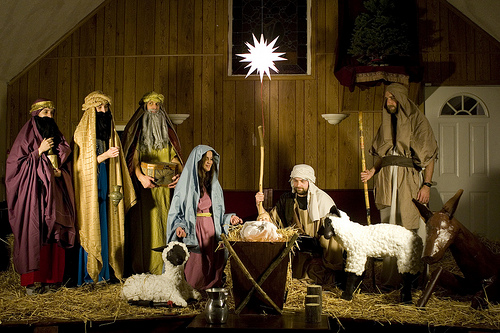This image is a highly detailed photograph of a live nativity scene staged to resemble the birth of Christ. The setting appears to be inside a wooden barn or stable, complete with a gabled roof with no ceiling and a wooden plank wall featuring a large window behind the scene. To the right, there's a modern wooden door with rectangular panels and a semicircular window at the top. The backdrop includes shiny reflective wooden floors scattered with straw to enhance the barn-like illusion.

At the center of the scene, baby Jesus lies in a manger filled with hay, with obviously fake sheep on either side. Mary, depicted as a woman with a bluish headscarf and a red robe, is seated beside the manger, gazing down at Jesus. Joseph stands to the right, alongside another man, both holding staffs. 

To the left stand the three wise men, distinguishable by their long robes and colorful, albeit cheap-looking, costumes and fake beards. The actors are positioned around the manger, immersed in the reenactment. Additional props like a toy sheep and a small donkey sculpture enhance the portrayal of the nativity, making the scene both vivid and detailed despite the artificial elements. 

This detailed setting, combined with the attire and positioning of the actors, creates an evocative recreation of the biblical nativity scene, capturing the essence of the traditional story in a theatrical context.